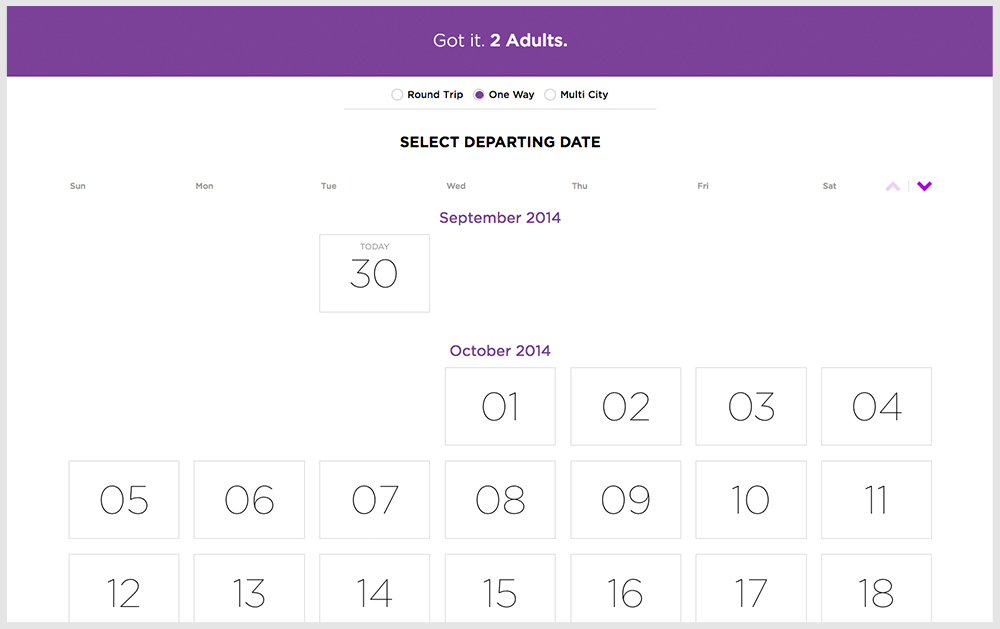The image features a travel booking interface with a dark purple border at the top. In the center of the border, it displays "Got it to adults." Below that, it lists three travel options: "Round Trip," "One Way," and "Multi-City." The "One Way" option is checked. 

Underneath, the text reads "Select Departing Date." The interface displays the days of the week from Sunday to Saturday, arranged from left to right. There is an upward-facing arrow and a downward-facing arrow, with the downward-facing arrow highlighted in purple. 

Below this, the date "December 30, 2014" is prominently shown. Further down, "October 2014" is indicated. 

In the main part of the interface, there is a calendar grid consisting of 18 white squares with gray borders. Each square is labeled sequentially from 01 to 18, starting from the top left and moving to the middle of the interface.